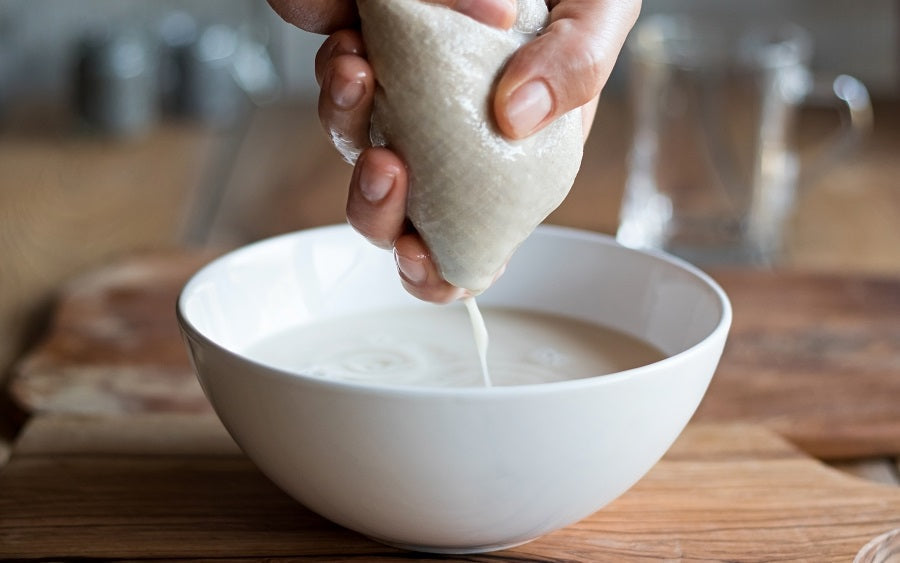In this color photograph, a Caucasian left hand with well-trimmed fingernails is shown squeezing a white liquid from a bag, possibly a plastic or pastry bag, into a white bowl. The hand appears wet from handling the bag. Positioned on a light brown wooden cutting board, the bowl is around halfway full of the whitish, cream-colored substance. The background is blurry but contains vague shapes of kitchen items. To the right, there is a glass mug or measuring cup, and on the left, there might be a loaf of bread, along with other indeterminate items. A hazy view of a wooden platter and additional glasses can be discerned further in the back.